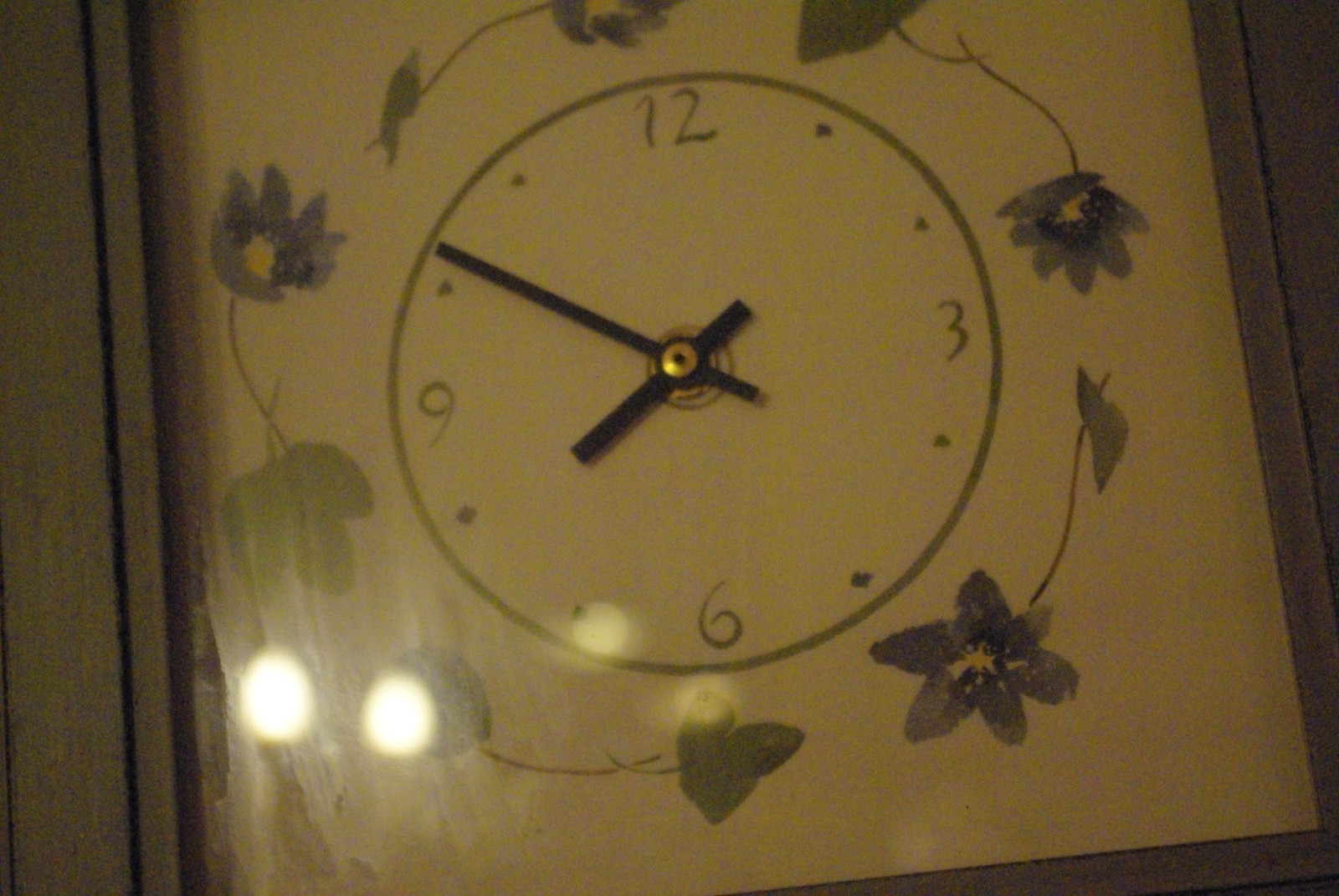The image showcases a hand-drawn clock on a yellowish piece of paper with a brown border. The background features brown wooden paneling on the left side and medium gray wooden paneling on the right. Overhead artificial lighting casts two white circles of light in the bottom left quadrant of the image.

The clock itself is depicted as a green circle with the numbers 3, 6, 9, and 12 positioned at their conventional points. Smaller dots mark the intervals between these numbers. The clock’s black hands indicate that the time is approximately 7:52. Surrounding the clock are artistic embellishments of purple flowers and green leaves, adding a touch of color and detail to the overall composition.